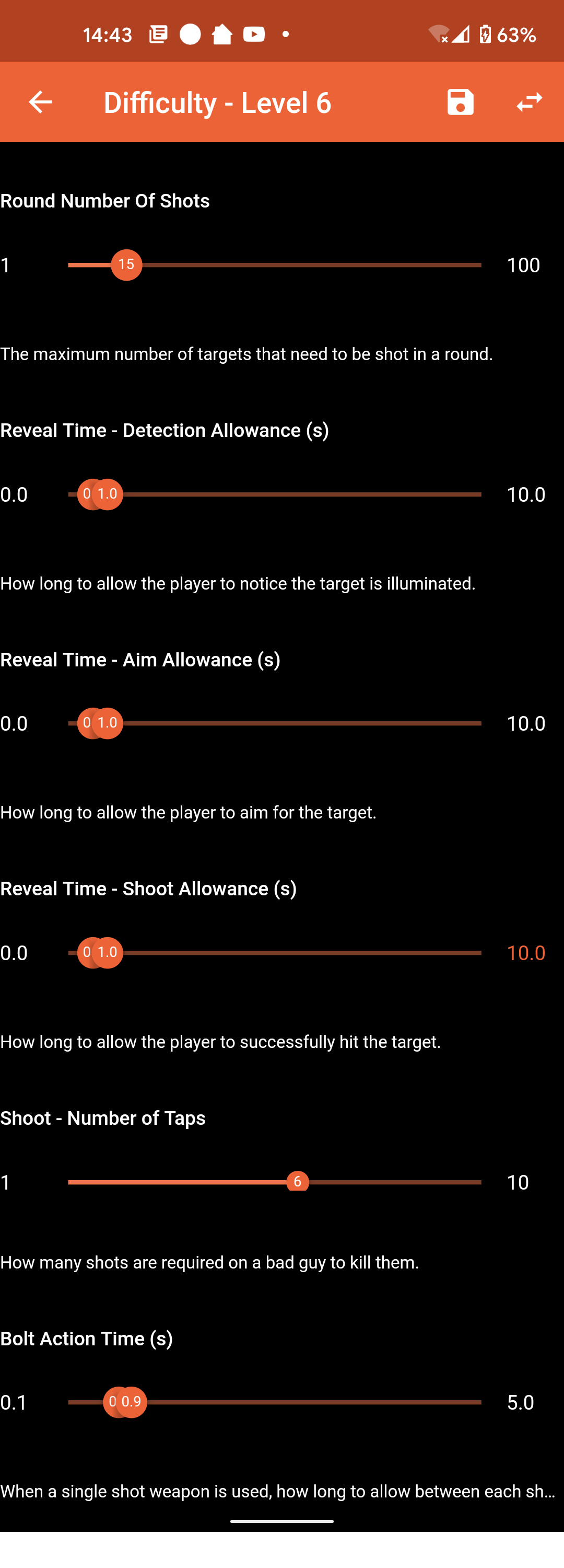This image is a portion of a screenshot, with the left side truncated and the overall view being long and narrow. At the top, the notification bar displays a brown-tan color. Directly below it, on the left, there's a left-pointing arrow accompanied by the text "Difficulty / Level 6." To the right of this text, there's an icon resembling a disc, with dual arrows - one above, pointing right, and one below, pointing left.

The majority of the screen beneath this section is black, populated by several slider buttons, each associated with specific controls:

1. **Number of Slots:** Adjusts the maximum number of targets that need to be shot in a round.
2. **Reveal Time:** Configures the duration allowed for the player to notice that a target is illuminated.
3. **Shoot Allowance:** Sets the time allowed for the player to hit the target with a single shot.
4. **Interval Time:** Determines the time permitted between each shot.

Each slider features a rounded design to facilitate user interaction.